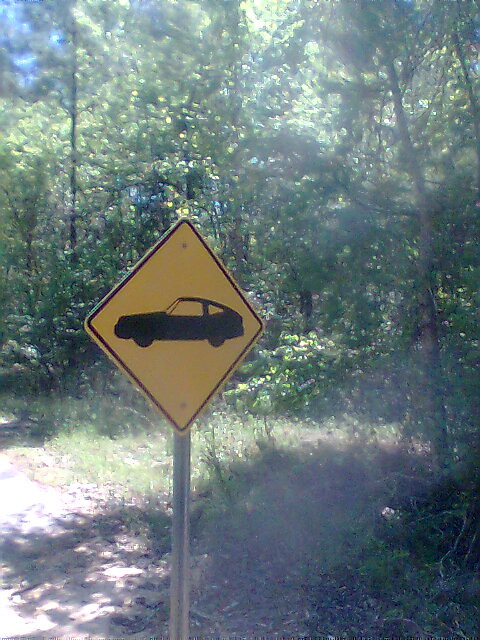In this image, a distinctive yellow, diamond-shaped traffic sign stands prominently on a typical gray metal pole against a backdrop of a mixed green and brown grassy field. The sign features a detailed, line-drawn silhouette of a two-door car facing left, complete with open areas for the windows, and bordered in black. Sunlight filters through the spindly trees in the background, casting hard shadows and creating bright spots on the leaves. The trees are largely green, suggesting it's summertime, with a hint of blue sky peeking through at the upper edge of the photo. The ground is littered with patches of dead grass, debris, and dirt, adding to the rustic and somewhat disarrayed scene. The sign itself is unusual and not immediately familiar, possibly resembling a more modern European design or a sports car icon.